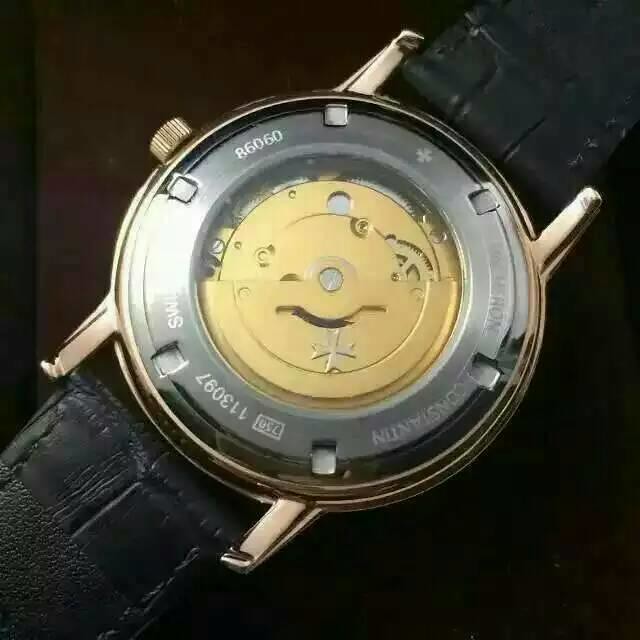A detailed close-up photograph captures what appears to be the back of a luxurious wristwatch. The watch features a circular gold frame around its face, encasing an inner ring of metal. Prominently displayed on this inner ring are the numbers "86060," accompanied by a small cross symbol. Etched text is also visible on the metal, although some of the inscriptions are obscured by glare. 

Around the wrist area, additional markings include the number "750" inside a rectangle, followed by the numbers "113097" and the letters "SW," which are partially washed out by the glare. The inner circle of the watch reveals intricate gold mechanisms, suggesting a view of its internal workings. The watch is equipped with gold brackets that connect to a black leather strap.

The background of the image is predominantly dark, with hints of red visible at the top, adding a subtle contrast. The entire bottom right half of the background remains pitch black, further emphasizing the watch as the focal point.